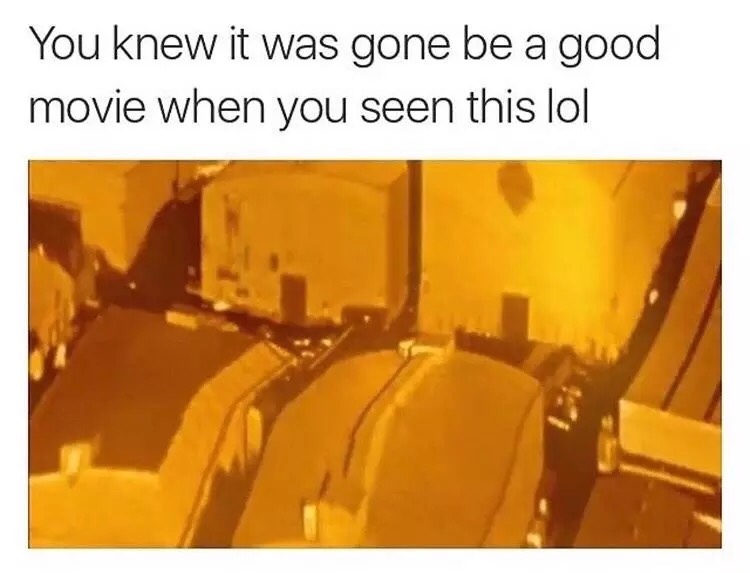The meme image features a sepia-toned still from the opening sequence of a classic movie, showcasing a top-down view of what appears to be the Paramount Studios lot in Los Angeles. The blurred picture, bathed in golden yellow hues, displays two rows of white buildings or warehouses lining a central road, evoking a sense of nostalgia. The upper part of the image contains black text on a white background that reads, "You knew it was going to be a good movie when you seen this lol," hinting at the familiar anticipation of a memorable movie experience marked by the iconic scene from the production company's introduction.